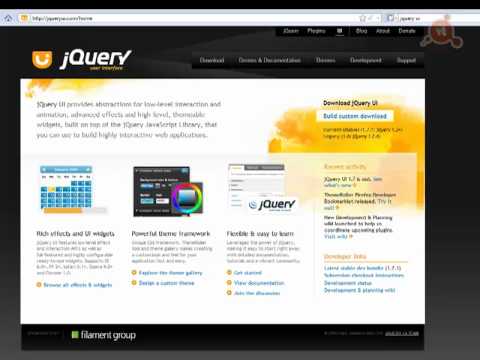This image depicts the homepage of the jQuery website, jQuery.com. At the top of the webpage, the URL is clearly visible, accompanied by a small orange square and an option to mark the site as a favorite. The entire background of the page is black, providing a stark contrast to the colorful elements on the site.

Prominently displayed at the top, the jQuery logo captures attention. The logo is an orange, purse-like shape containing a white, stylized "U" shape, which resembles a small spark or flame. This logo is followed by the text "jQuery," where the 'j' is lowercase and the 'Query' starts with a capital 'Q' but the 'uery' is in lowercase, all written in white.

Beside the jQuery logo and text, there are several options presented, although they are somewhat difficult to discern due to the blurry quality of the image and the small font size against the black background.

Further down, the page provides more information about jQuery, including an option to download it. This section elaborates on how to use jQuery, highlighting its benefits and use cases. It explains that jQuery is a JavaScript library designed to simplify coding, making it more efficient to write scripts. The central portion of the page features various images and graphical representations that illustrate the capabilities and applications of jQuery, although these too are affected by the blurriness of the image.